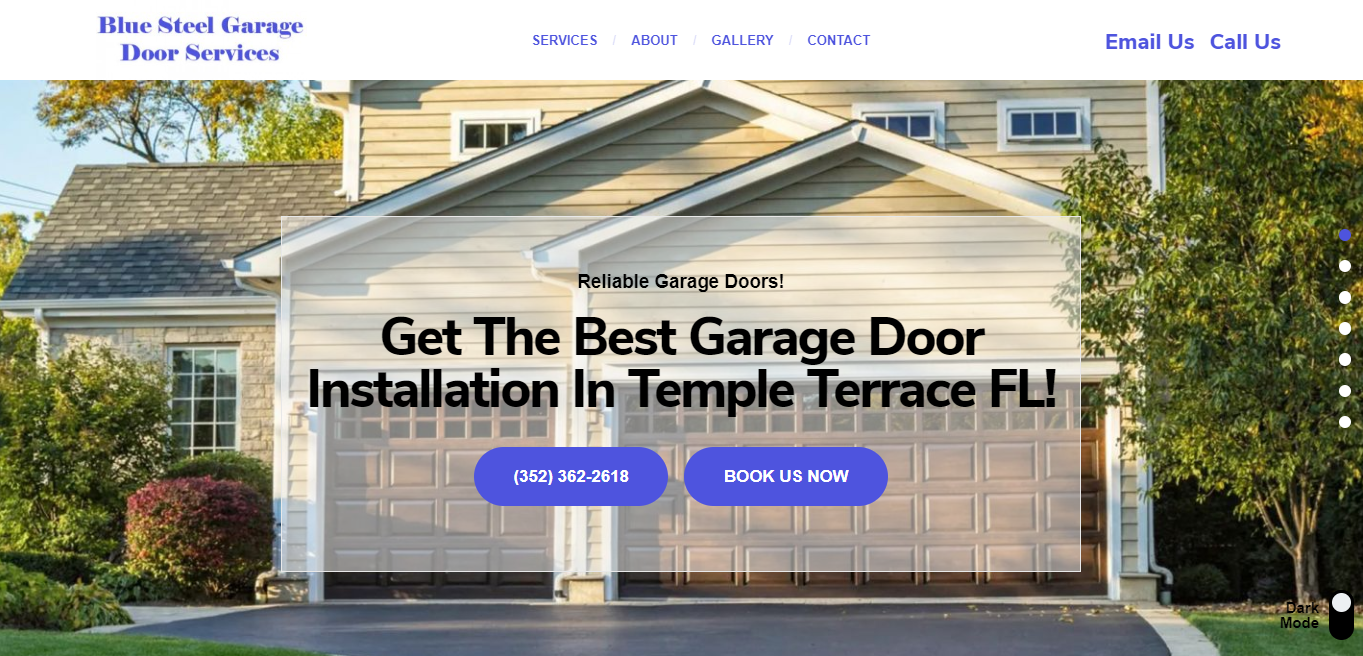A vibrant, cheerfully detailed image showcases a picturesque two-story house in Temple Terrace, Florida. The charming home, exuding warmth with its soft yellowish hue complemented by crisp white trim, features an aesthetically pleasing combination of brick and siding. A prominent two-car garage proudly displays a message for "Blue Steel Garage Door Services," urging viewers to "Get the best garage door installation in Temple Terrace, Florida," complete with a visible contact number. The house, possibly containing upstairs bedrooms, is framed by well-maintained shrubs and leads onto a pristine asphalt driveway. Bathed in the glow of a brilliant blue sky and surrounded by lush greenery, the scene captures the essence of an idyllic, upscale Floridian neighborhood. The ad encourages potential customers to explore their gallery and contact them, boasting a reputation for beauty and quality in their services.